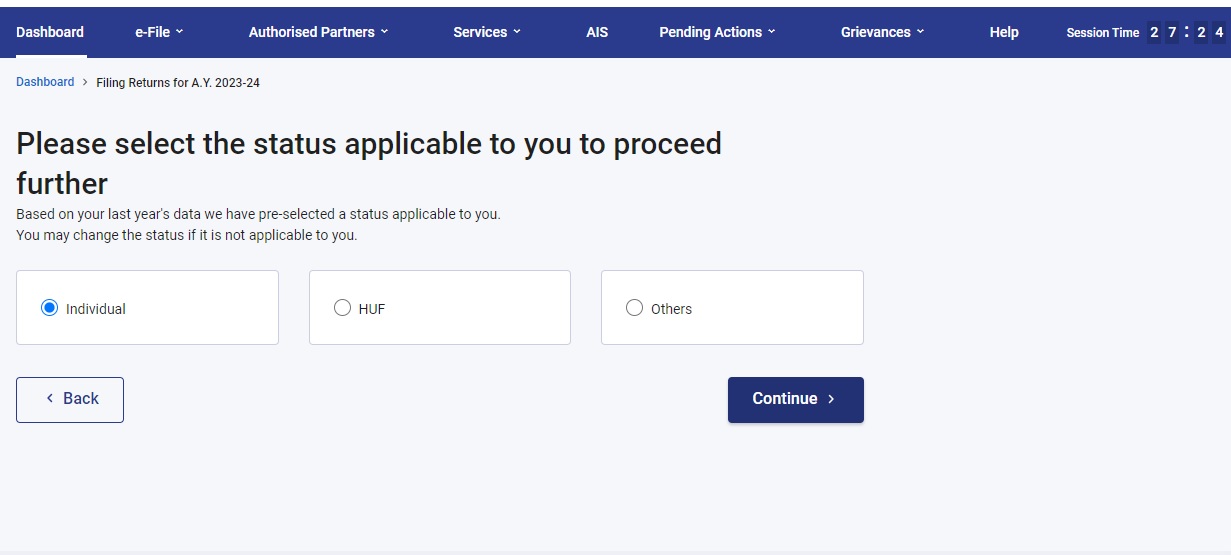A computer screen displays the initial page of a do-it-yourself tax filing software. At the top of the screen, a blue bar contains various menu options including "Dashboard," "e-File," "Authorized Partners," "Services," "AIS," "Pending Actions," "Grievances," "Help," and "Session Time." The current session time is displayed as 27:24, though it is unclear whether this represents minutes and seconds or hours and minutes.

The main content of the screen indicates that the user is filing returns for the initials "A.Y." for the tax year 2023-2024. A prompt requests the user to select their applicable status to proceed, noting that the system has pre-selected a status based on the previous year's data. The selectable options include "Individual," "HUF," and "Others," with "Individual" currently selected.

An instructional message advises the user that they may change their status if the pre-selected option does not apply to them. At the bottom of the page, there are buttons to continue or navigate back, suggesting the user is at the beginning stages of completing their tax return.